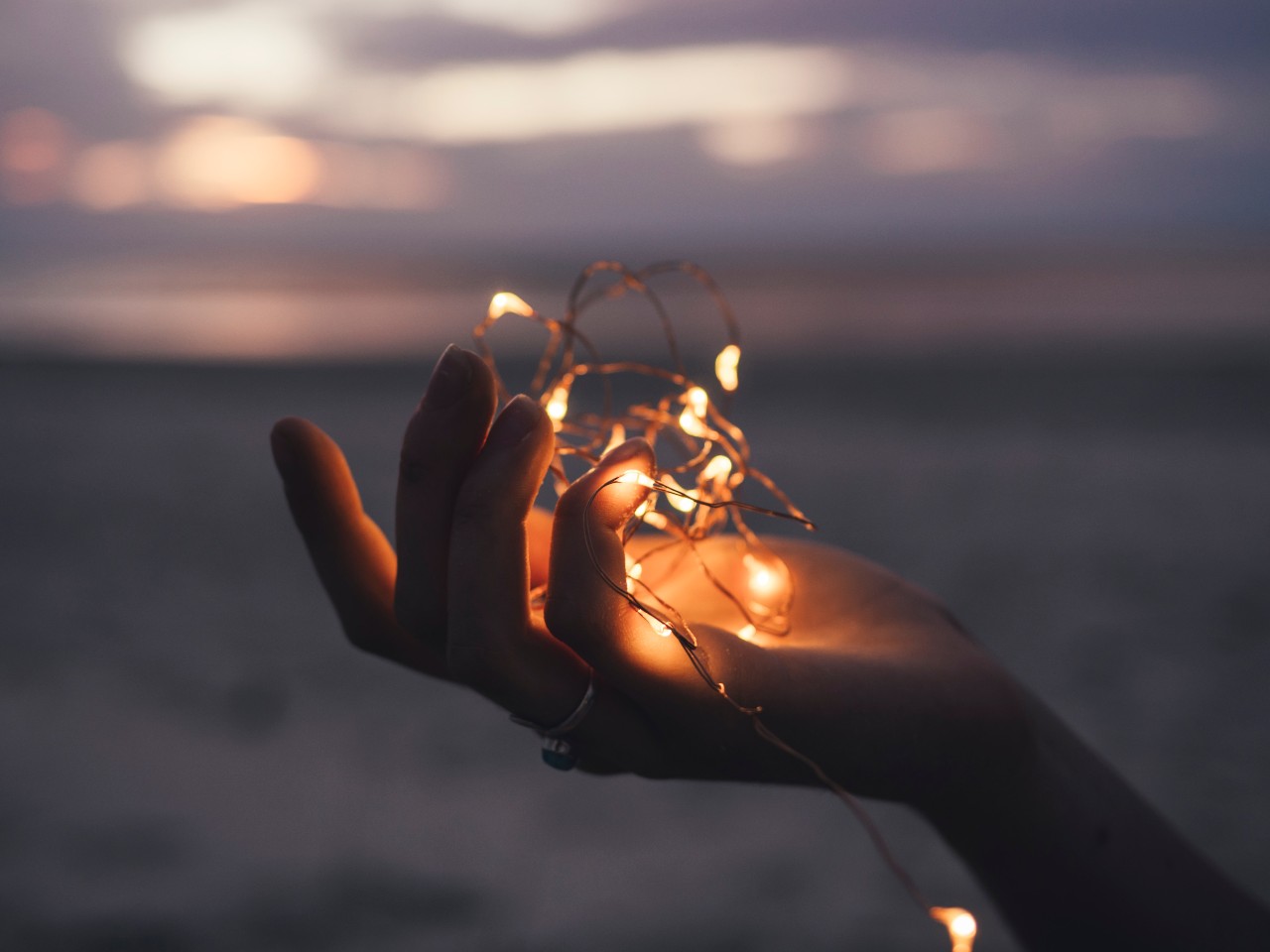This image captures a serene beach scene at what appears to be sunset. Front and center, a hand stretches outward, delicately holding a bundle of thin wire string lights. The lights, small and white or yellow, cascade down the wrist and forearm, which is cropped mid-forearm in the frame. The soft glow of the lights illuminates the creases and contours of the hand, including a silver and blue ring adorning the index finger. The background, although out of focus, suggests a tranquil beach setting with sandy shores and distant waters blending into the horizon. The lighting may have been enhanced to accentuate the warmth emanating from the string lights, adding a gentle, ethereal quality to the composition. The sky hints at the day's end, with subtle hints of clouds and the fading light of the sun giving the scene a peaceful twilight ambiance.